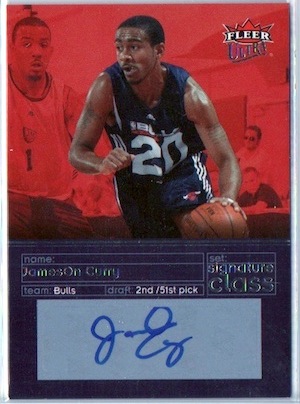The image depicts a basketball trading card featuring the player JamesOn Curry wearing a dark blue jersey with the number 20. The word "Vols" is displayed above the number on the front of his tank top. The top right corner of the card bears the logo and name of the company, F.L.E.A.R. The card background consists of a red and black photo of a basketball game, with a cut-out action shot of Curry dribbling a basketball superimposed in the middle. The bottom third of the card provides information about Curry, including his name, team, and draft details—specifically noting that he was the 51st pick in the second round. Beneath this information, in a teal blue square, is Curry's signature written in blue pen.